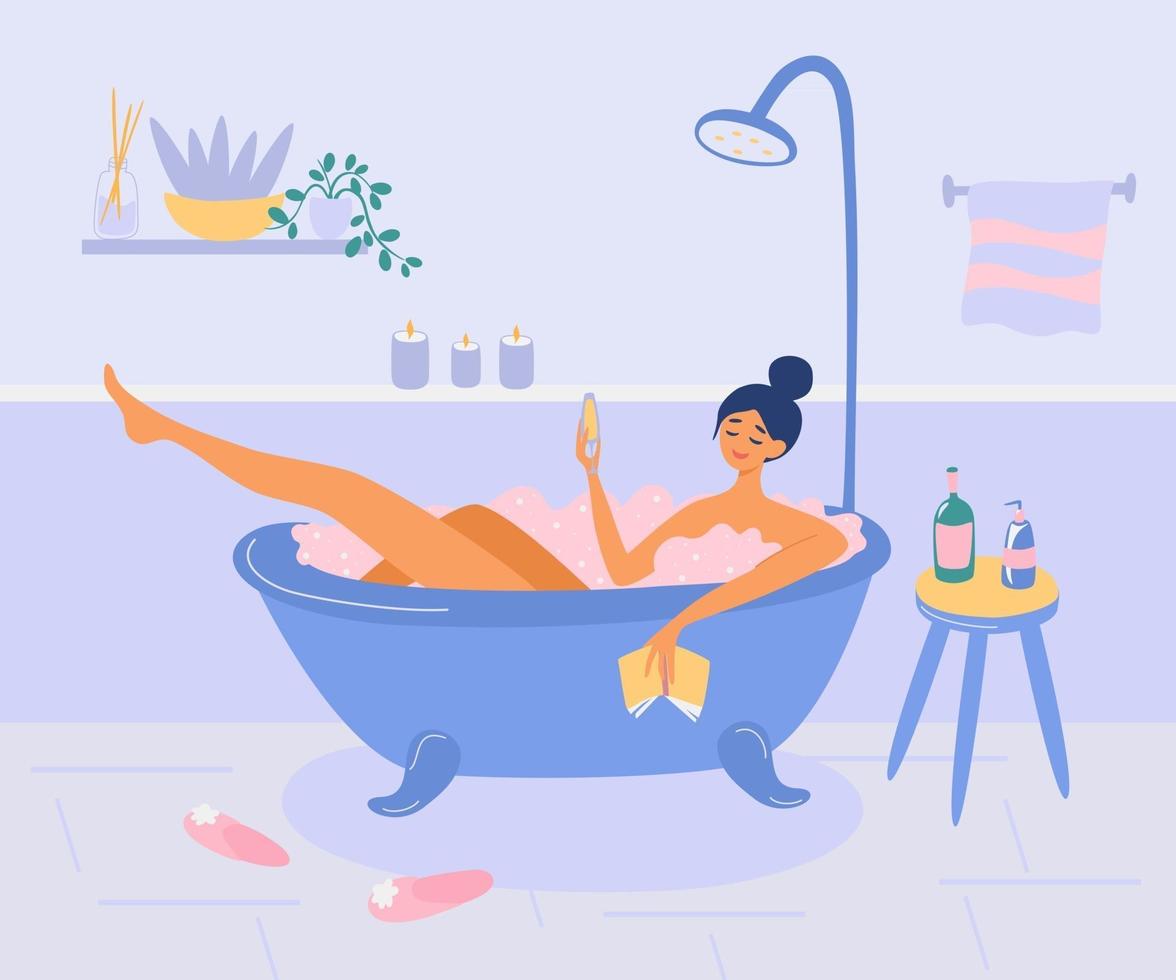The illustration depicts a woman with dark hair swept up into a bun, luxuriating in a blue clawfoot bathtub filled with pink foam. She has one leg extended out of the tub and is holding a book with a gold cover in one hand and a glass of wine in the other, all while smiling and appearing very relaxed. Surrounding her are various items: a pair of pink slippers set beside the bathtub, a stool on the right holding a champagne bottle and a soap dispenser, and a light lavender and pink towel hanging from a towel bar in the top right corner. The walls of the bathroom are painted blue. A shelf on the left side holds sticks in a bottle and two potted plants with green and blue leaves. Additionally, the ledge behind the bathtub displays three lit candles, contributing to the calming ambiance of what appears to be a stylist's bathroom.